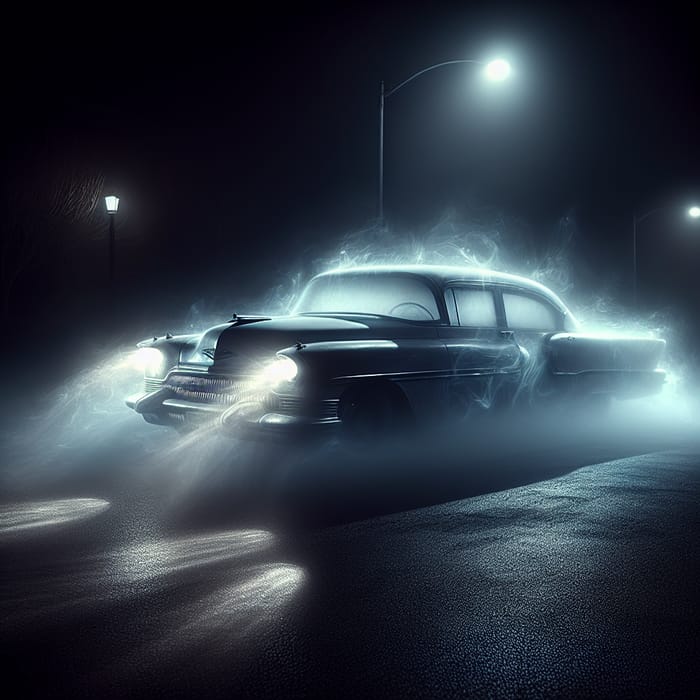In this atmospheric, night-time photograph, an eerie, fog-enshrouded 1950s-style car is captured on a dark asphalt road. Positioned centrally, the vehicle is flanked by a trio of streetlamps whose beams cut through the dense mist. Directly above the car, one of these lamps casts an ethereal glow, while the others loom in the obscured background. The car, possibly blue or gray, has its headlights on, their beams piercing the fog and casting reflections on the wet pavement and the car itself. Through the hazy windows, only the vague outline of the steering wheel is discernible, enhancing the mysterious vibe, as there appears to be no driver. The grille at the front of the car resembles tightly packed teeth, adding to the spooky, almost sinister aura of the scene. To the left, partially illuminated by the streetlight, a tree emerges from the darkness, contributing to the photograph’s unsettling ambiance.